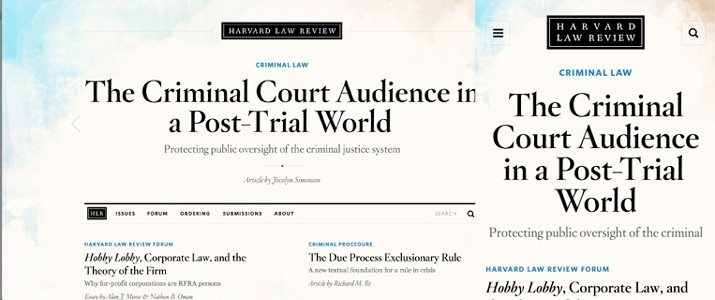The image features a webpage preview of the Harvard Law Review, showcasing both desktop and mobile formats side by side. At the top, the desktop version prominently displays "Harvard Law Review" followed by headers such as "Criminal Law" and "The Criminal Court Audience in a Post-Trial World: Protecting Public Oversight of the Criminal Justice System," an article whose author's name is illegible due to small text. Below, there is a black navigation bar with options like "Help," "Issues," "Forum," "Ordering," "Submissions," and "About," alongside a search icon.

Further down, there is another headline in blue text: "Harvard Law Review Forum" with the title "Hobby Lobby, Corporate Law, and the Theory of the Firm." To its right, another section reads "Criminal Procedures," with a subsequent title "The Due Process Exclusionary Rule." 

On the right side of the image is the mobile version of the same page, with the same content but formatted for mobile viewing. It includes the Harvard Law Review logo, the sections on Criminal Law and the post-trial world, and the same articles and forum titles. The mobile format also features a magnifying glass in the upper-right corner for search functionality and a hamburger menu icon in the upper-left for navigation. The background of the webpage showcases an open sky with scattered clouds, adding a serene backdrop to the academic content.